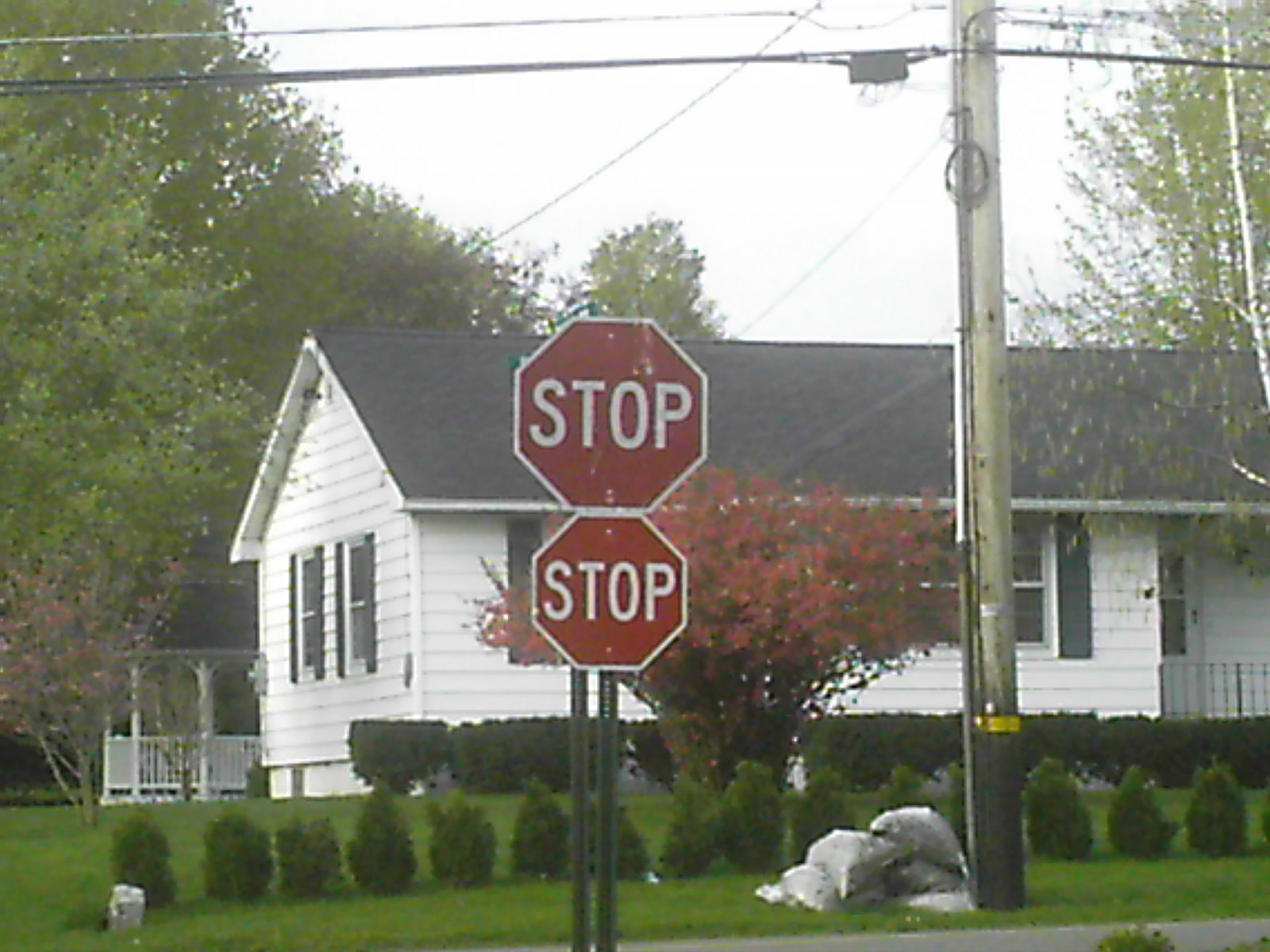This image captures a picturesque suburban corner featuring a white ranch house with black shutters and a black roof, partially visible in the center backdrop. The house boasts a white front door with a small railing and is flanked by neatly trimmed bushes. A vibrant red-leaved tree stands in front of these bushes, while smaller evergreen saplings are planted between the road and the red tree. Dominating the foreground are two stop signs mounted on green poles, with the larger sign positioned above the smaller one. Adjacent to the stop signs stands a telephone pole wrapped with wires extending left to right, and sandbags or piles of leaves are stacked at its base. The lush, green lawn extends from the house to the road, enhancing the serene ambiance of the scene. In the yard's corner and slightly set back, there is a quaint white gazebo with a black roof surrounded by tall green trees. Nearby, a birch tree sports its distinctive white bark, and a mix of another orange and pink flowering tree adds splashes of color to the landscape. The horizon reveals more greenery and a cloudy sky, adding depth to this idyllic neighborhood snapshot.